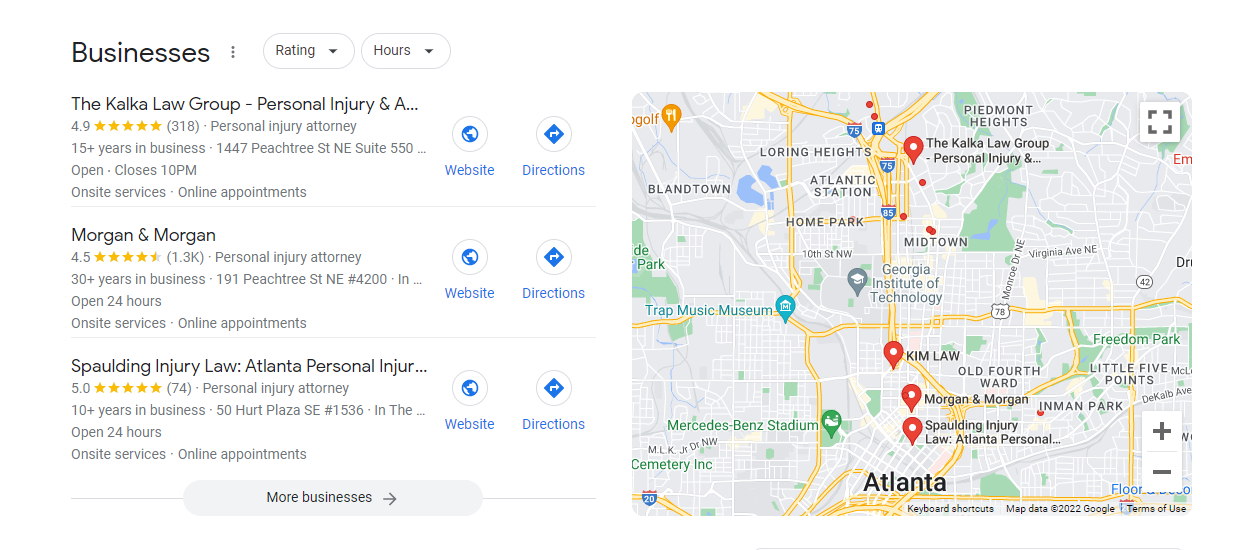The image showcases search results for personal injury attorneys from Gopi. The interface prominently features the word "Businesses" at the top left corner. The background is white, and the text is in black. 

**Listings:**
1. **The Calcalo Group Personal Injury Attorney**
   - **Rating:** 4.9 stars, rated by 2,018 people
   - **Experience:** 15+ years in business
   - **Address:** 1447 Peachtree Street
   - **Hours:** Closes at 10 PM
   - **Services:** On-site service, online appointment
   - **Buttons:** “Website” and “Directions” in blue
   
2. **Morgan & Morgan Personal Injury Attorney**
   - **Rating:** 4.5 stars, rated by 1.3K people
   - **Experience:** 3+ years in business
   - **Address:** 191 Peach Street, NE H4200
   - **Hours:** Open 24 hours
   - **Services:** On-site service, online appointment
   - **Buttons:** “Website” and “Directions” in blue
   
3. **Spaulding Injury Law, Atlanta Personal Injury Attorney**
   - **Rating:** 5 stars, rated by 74 people
   - **Experience:** 10+ years in business
   - **Address:** 50 Hard Plus SA, Number 1536
   - **Hours:** Open 24 hours
   - **Services:** On-site service, online appointment
   - **Buttons:** “Website” and “Directions” in blue

**Additional Elements:**
- Yellow star ratings for each business.
- A map is located on the right side of the image displaying the location in Atlanta.
- Drop-down buttons for additional filters such as ratings and business hours.

Overall, the image provides a detailed directory of top-rated personal injury attorneys in Atlanta with essential business details and easy navigation options.